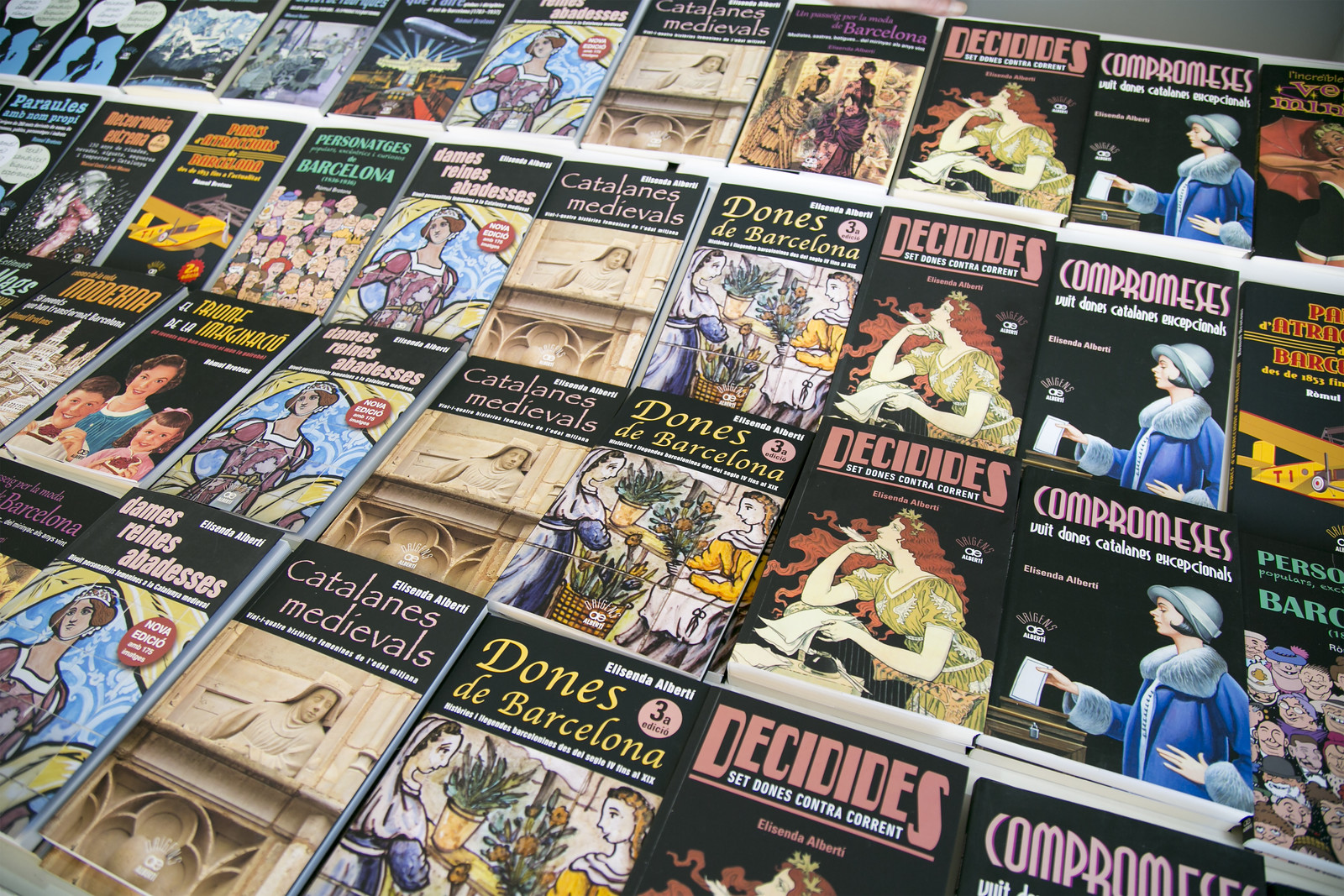The image showcases an overhead view of multiple rows of books neatly aligned in a horizontal rectangular frame reminiscent of a magazine rack. Each book's front cover is visible, revealing a variety of titles and vivid cover illustrations primarily featuring women from different historical periods. The titles of the books include recurrent appearances of “Decidides,” “Compromises,” “Dones de Barcelona,” “Catalanes Medievales,” and “Damos Reyes Abadesis.” 

In the top left corner, we see partially visible solid gray, suggesting a wall beyond the bookshelves. Among the covers, the designs vary widely, with one displaying a yellow airplane, while another features an astronaut in a red suit. Titles like “Decidides” include an Art Deco image of a woman gazing wistfully over a piece of paper, while “Compromises” showcases a woman in 1920s attire. Covers for “Dones de Barcelona” and “Catalanes Medievales” present women adorned in long dresses, old-fashioned coats, and hats, reflecting styles from medieval times to the 1950s. The color palette spans across pinks, yellows, blacks, oranges, and purples, with each row meticulously repeating the titles, indicating possibly multiple copies or different editions. 

Prominently, the covers display rich historical and artistic detail, including illustrations of regal women and nun statues, adding depth and intrigue to the overall composition. At the far left-hand top corner, a book titled “Paralysis” features two blue silhouetted figures, breaking the pattern of historical imagery with its modern silhouette. Each book cover contributes to a colorful and historically evocative tableau.